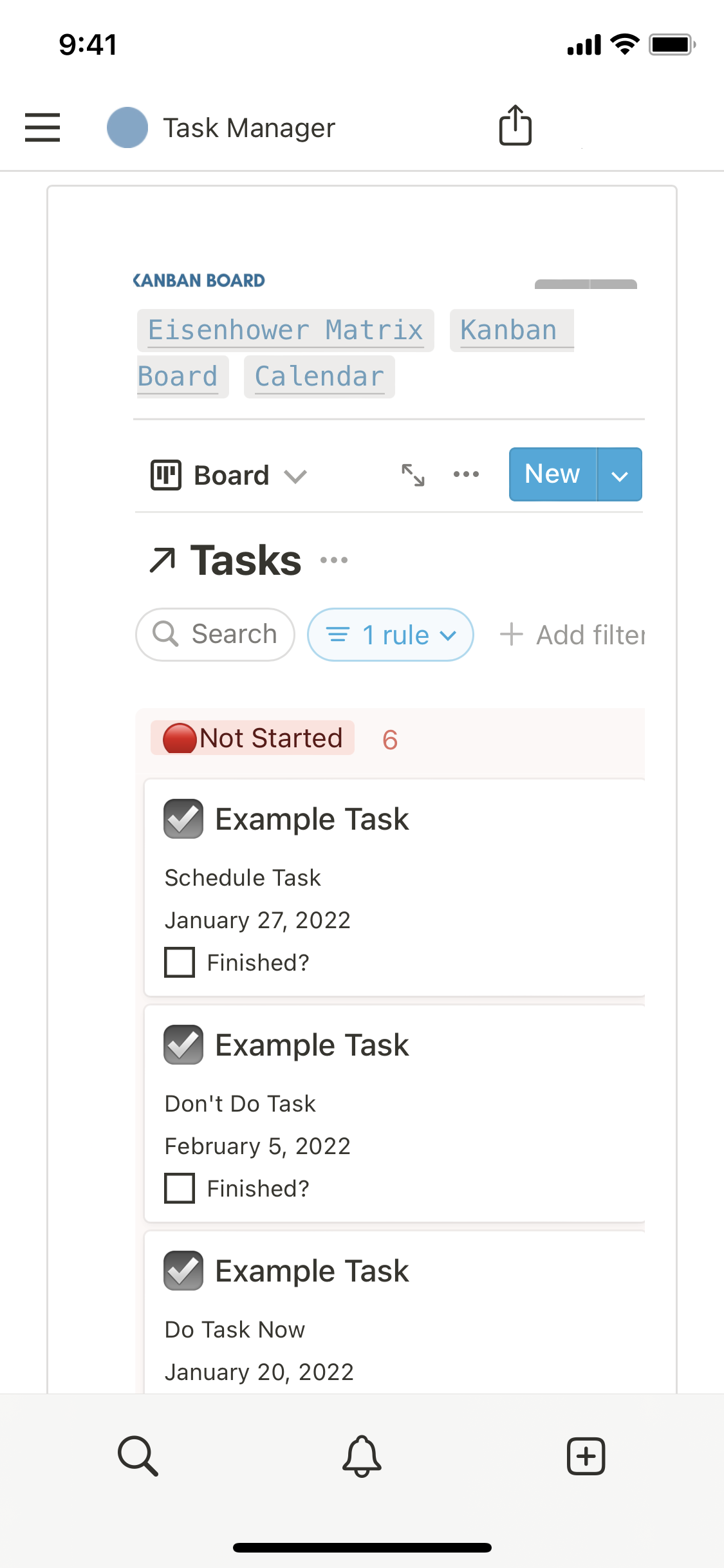**Detailed Caption:**

The image depicts the interface of a website displayed on a smartphone. At the top of the screen, the time reads "9:41", without indicating whether it is AM or PM. To the right, the status bar shows full battery, phone signal bars, and Wi-Fi connectivity.

On the upper left corner of the screen, there are several menu buttons. Immediately next to these is a blue-filled circle labeled "Task Manager." Just beside it, there's an upload icon, which is followed by a horizontal line.

Beneath this line, there's a box containing multiple elements: 
- "Kanban Board Eisenhower Matrix"
- "Kanban Board Calendar"

Below this box appears the word "Board" accompanied by a downward arrow, suggesting a dropdown menu for additional options. Adjacent to this, there's a "New" button, which, when pressed, likely reveals more functionalities.

Further down the interface, there is a "Tasks" heading, under which you find a search bar labeled "Search" and an "Add Filter" option. Below these, a red button with red text displays "Not Started 6".

The task list begins with:
1. An "Example Task" with a white check mark inside a black box, scheduled for January 27, 2022. A checkbox beside this task allows users to mark it as completed.
2. A second list item labeled "Don't Do Task," dated February 5, 2022.
3. A third "Example Task," which adds to the series of tasks listed. 

The overall layout of the interface suggests a well-structured task management system designed to enhance productivity.